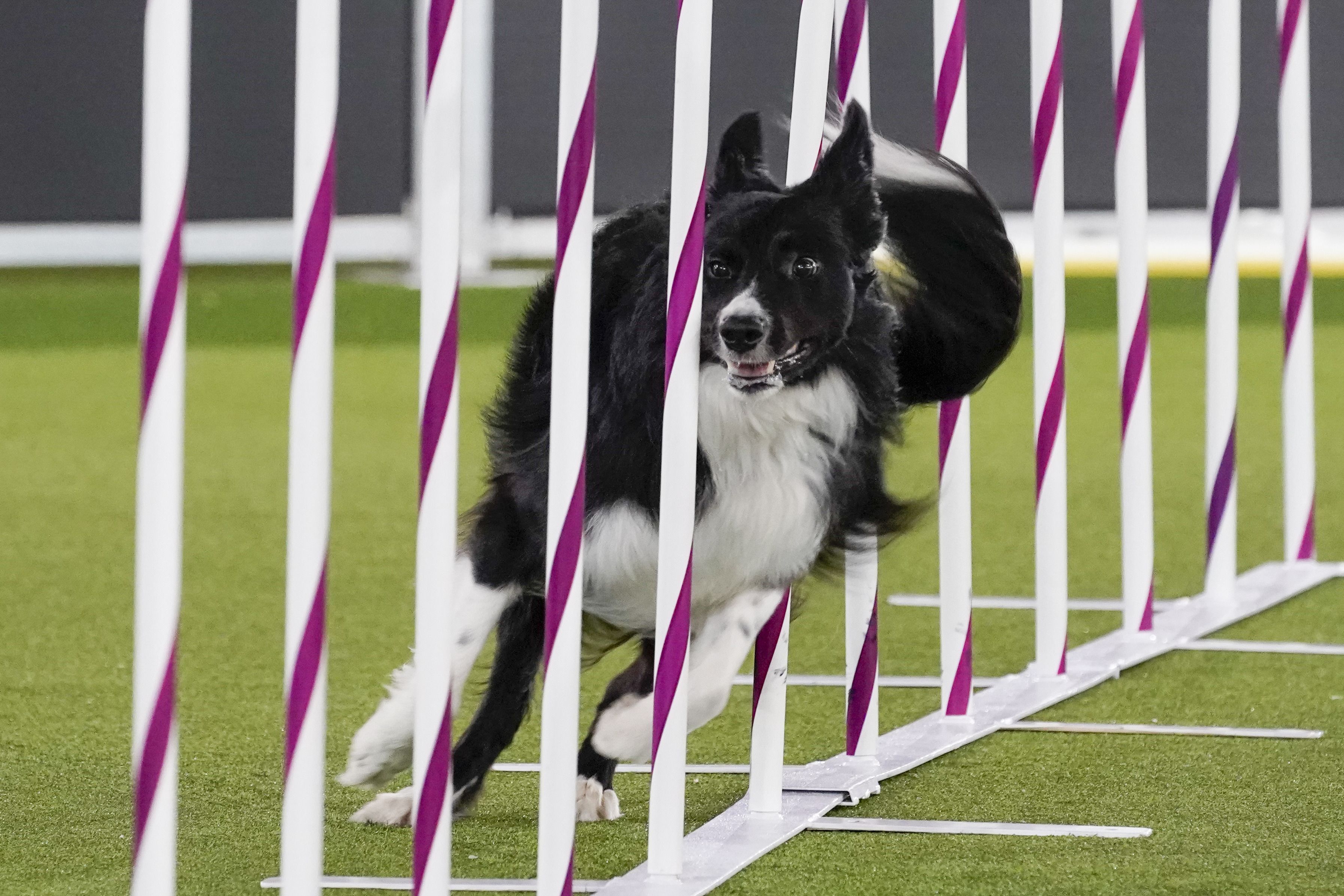This detailed digital photograph captures a dynamic moment of a black and white dog energetically navigating an obstacle course, likely part of a dog show or event. The horizontally aligned rectangular image prominently features a series of white vertical poles adorned with purple diagonal stripes, which the dog is skillfully weaving through. These poles are attached to a narrow white rectangular base, positioned diagonally from the upper right to the center left of the frame. The setting appears to be a football or soccer field covered in short green synthetic turf, with white tape marking the course.

The dog, mid-action with its mouth slightly open, has striking features: pointy black ears, a long black tail tipped with white, and a predominantly black coat with a white underside and snout. Its front paws are white, while the back paws are black with distinctive white toe beans. Its eyes are brown, adding a touch of depth and expression to its determined face. The backdrop of the image includes a grey wall at the top, providing a neutral background that makes the vivid colors and action in the foreground stand out.